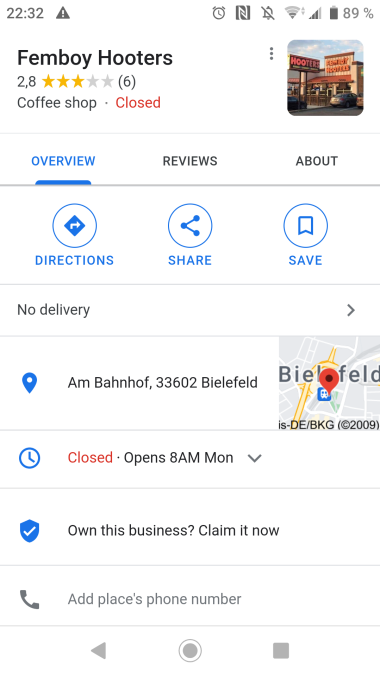This image is a detailed screenshot from a smartphone displaying a Google Maps business listing for an establishment humorously named "Femboy Hooters." 

In the status bar at the top of the phone screen, the time reads 22:32, alongside indicators for carrier signal strength and a battery with 89% charge.

The listing shows that "Femboy Hooters" has a 2.8-star rating based on 6 reviews and is currently marked as closed, highlighted in red text. Accompanying the listing is an image featuring a typical Hooters sign, suggesting an illusory or altered photograph to match the joke business name.

The interface includes three main tabs: Overview, Reviews, and About, with the Overview tab currently selected and highlighted in blue. Below these tabs, large circular buttons offer various actions such as getting directions, sharing the listing, or saving it.

The listing notes that delivery is not available from this location. The provided address, "AMBAHNHOF33602BELILIFELD," appears to be fictitious or a possible reference to something unknown, as it does not resemble a legitimate address.

A small map snippet displays a red pin marking the supposed location in an area referred to as Belilifeld, further casting doubt on its authenticity. The business status shows it is closed and includes additional details in red text indicating it will reopen at 8 AM on Monday.

Towards the end of the listing, there is a prompt encouraging business owners to "Claim this business!" and take control of the listing. Additionally, there is a phone number icon typically seen in Google Maps business listings but no actual phone number listed here. Based on the humorous nature and various inconsistencies, it strongly suggests that this is not a real business but rather a satirical creation that has now been captured in a screenshot.